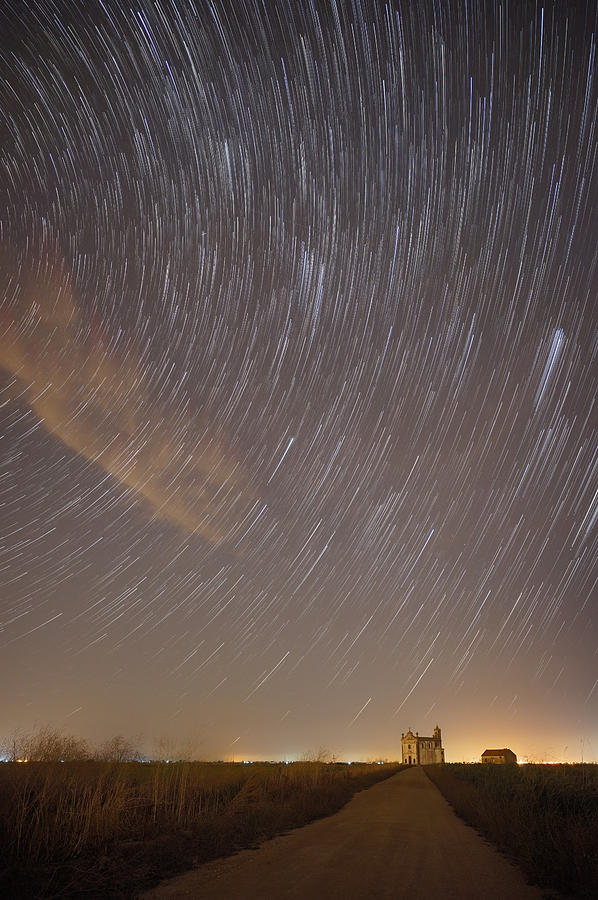An eerily atmospheric night scene captures a long dirt road stretching into the distance, flanked by fields and brush on either side. At the end of the road, a small castle-like structure looms, accompanied by a smaller building nearby. The dark sky above is studded with stars, their paths traced in a time-lapse, suggesting an ethereal beauty. A faint glow encircles the buildings, contrasting with the deep blues and blacks of the night, reminiscent of an AI-generated landscape. The entire scene has an almost surreal quality, with thin, white streaks breaking through the sky and a faint cloud lingering to the right, making the setting appear simultaneously familiar and fantastical.